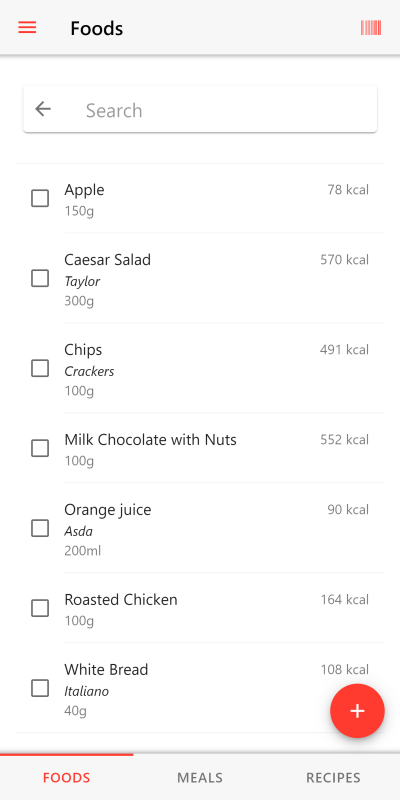In this screenshot, a variety of food items are presented on a user interface. The upper section of the image includes navigational and identification elements. At the top left, the word "foods" is displayed in black text, accompanied by three red horizontal bars stacked on top of each other, which may indicate a menu or options button. On the top right, a red barcode-styled logo adds a distinctive design element. This top section rests on a grayish background.

Below this header, there is a rectangular search area featuring the word "search" in gray text on the left side, with a left-pointing arrow icon even further to the left, also in gray.

Centrally, the main content shows a selection of seven different food items arranged in a structured format. These items are listed as follows:
1. Apple
2. Caesar Salad
3. Chips
4. Milk Chocolate with Nuts
5. Orange Juice
6. Roasted Chicken
7. White Bread

Finally, at the bottom of the image, three categories are displayed: "foods," "meals," and "recipes." The current selection, "foods," is highlighted in red to indicate it is the active category.